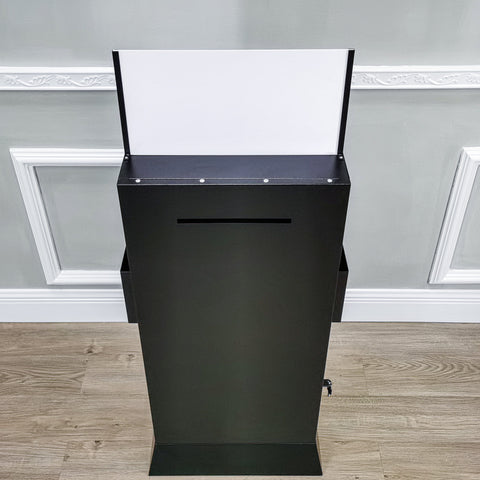The image features a perfectly square photograph depicting a household appliance or tool, centrally positioned against a medium-shade wooden floor occupying the bottom 40% of the image. Above the floor, a white footboard separates it from a gray wall accented with white trim. The focal point of the image is a sleek, rectangular appliance or tool, black at its base. Extending from its sides are two black bars, flanking a central white section that could potentially be a small projector screen or another functional component. At the top of the white section, four silver screws are visible, lined up horizontally. Directly below the screws is a cut-out slot, likely purposed for sliding in letters or materials. The image is devoid of any people or text, allowing for an unobstructed view of the object and its surrounding environment.